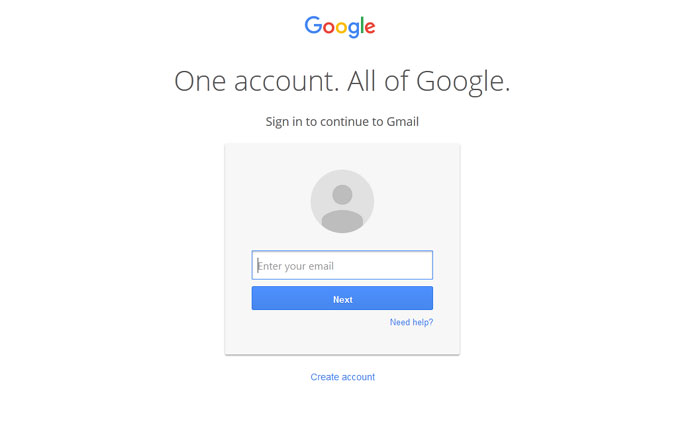The image depicts a screenshot of a Google sign-in page. Centrally positioned at the top is the Google logo, showcasing its characteristic colors: blue, red, yellow, and green. Below the logo, in larger font, the text reads "One account. All of Google." In a smaller font beneath it, the text instructs users to "Sign in to your Google Account" with their Gmail credentials.

Centered on the page is a gray rectangle containing a grayed-out, circular profile picture placeholder, indicating where a user's photo would appear. Below this placeholder is a long, white rectangular input box meant for users to enter their email addresses, with a blinking cursor positioned at the starting point of the input field.

Further down, there is a blue rectangular button with the word "Next" displayed in white font. To the right of this button, in blue font, is the link "Need help?" accompanied by a question mark. Outside of the input box area, at the bottom, another blue link reads "Create account," guiding new users to set up a Google Account.